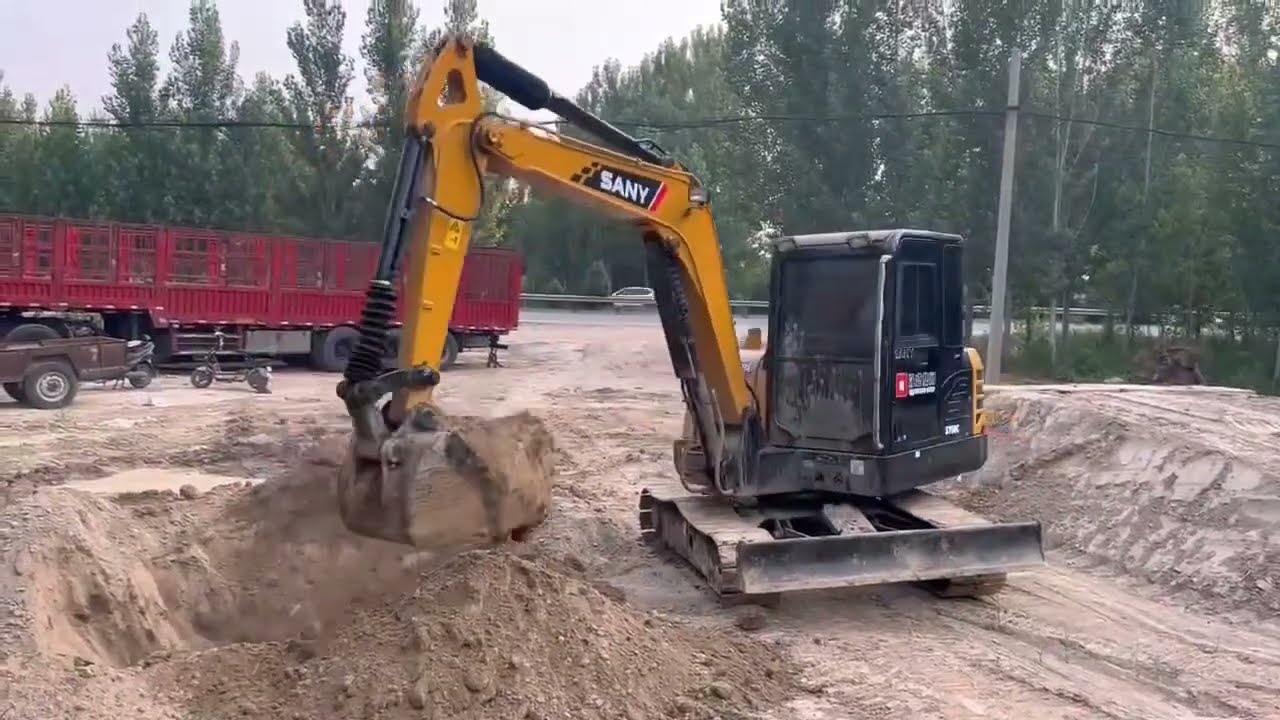In this image, we see a busy construction site under a gray, overcast sky. The central focus is a SANY-branded mini excavator. This robust machine features a black cabin and dusty rollers, with a prominent yellow arm extending to the left. Its bucket is filled with a large lump of brown dirt, revealing a freshly dug hole beneath. Surrounding the excavator, the ground is largely composed of loose brown dirt, accentuating the earthy tones of the site. 

In the background, a vast expanse of green trees stretches from the left to the right, creating a vivid natural backdrop. A gray telephone pole and a road are also visible, adding to the industrial setting. On the left edge of the image, there’s a brown pickup truck with what appears to be a motorized scooter or motorcycle behind it. Additionally, there is a long red trailer bed truck positioned behind the excavator. Overall, the image captures a dynamic moment at an outdoor construction site dominated by muted, earthy colors and the diligent activity of the mini excavator.